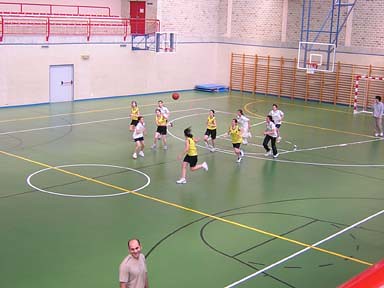This photograph captures a dynamic scene in a gymnasium where a women's basketball game or practice session is underway. The gym features a green basketball court adorned with a variety of lines in yellow, white, and black, indicating different sports activities. The upper section of the gym's walls is constructed of reddish brick, transitioning to a tan lower section trimmed in blue, with a white door visible in the upper left.

On the court, ten women are divided into two teams. One team wears yellow tank tops paired with black shorts, while the other team wears white tops with black shorts, and one player is in black pants. The players are energetically running towards an orange basketball that is mid-air, possibly indicating an active play. 

In the mid-right of the image, a person in khaki pants and a long-sleeved shirt, likely a coach, is engaged in watching the game. In the foreground, closer to the center, another man with a balding head dons a beige t-shirt and is facing away from the players, seemingly conversing with people off-camera.

The gymnasium also contains wooden fitness bars along the walls and a non-basketball goal, such as a soccer or hockey goal, positioned against the wall, adding to the multifunctional use of the space. The ceiling-mounted basketball hoop is partially visible in the upper right corner, reinforcing the sports setting.